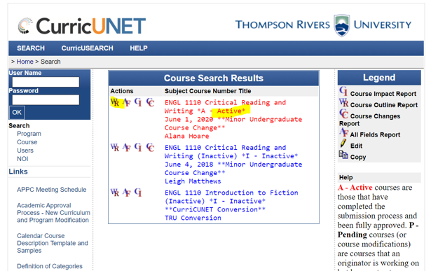The screenshot displays the Curricunet website interface associated with Thompson River University, prominently noted in the top-left corner. A blue horizontal navigation bar spans across the top of the screen, with the words "CurricuSearchHelp" clearly marked in white. Below this band, there are options and fields for "Home," "Search," "Username," "Password," and an "OK" button, with the input fields in white and the text in white as well, enclosed within a blue rectangle.

Further down, there is a navigation sidebar that lists various sections: "Search," "Program," "Course," "Users," and "NOI." Under this section, there are additional links titled "APPC," "Meeting Schedule," "Academic Approval Process-New Curriculum and Program Moderation," "Calendar Course," "Description Template," and "Samples," alongside a partly obscured text likely defining these terms.

Dominating the central portion of the webpage is the "Course Search Results" section distinguished by another blue bar with white text. Below this, columns are labeled with "Actions," "Course Subject," "Course Number," and "Title." The results displayed include an entry "WRAFCICC," linked to "English 1110" titled "Critical Reading and Writing." The status "AACTIV" is highlighted in yellow and shown in red font, drawing immediate attention.

The overall layout is characterized by a consistent use of blue and white color themes with highlighted elements for emphasis.